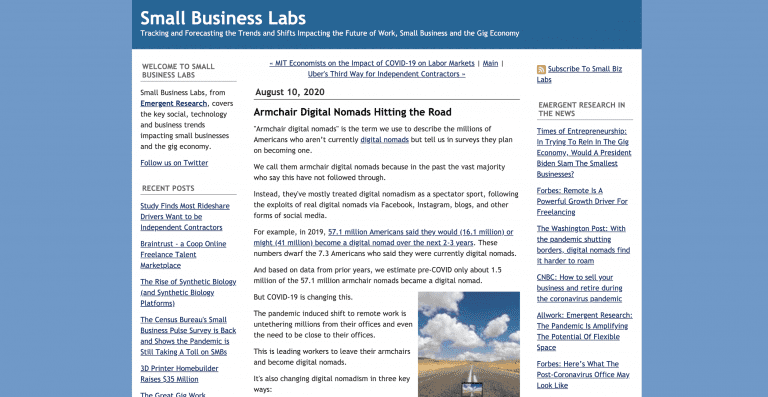In this image, we see a screenshot of a web page prominently featured in the upper left corner. The header reads "Small Business Labs," with a tagline that says "Tracking and forecasting the trends and shifts impacting the future of work, small business, and the gig economy." An article dated August 10, 2020, titled "Armchair Digital Nomads Hitting the Road" is displayed alongside a few paragraphs of text.

Running vertically down the left side of the page is a section labeled "Welcome to Small Business Labs," followed by another section called "Recent Posts," which contains several underlined article links. On the right side, near the top, the page invites users to "Subscribe to Small Biz Labs," with a subsequent section titled "Emergent Research in the News," also featuring numerous underlined article links.

The layout is accented with thick blue colored blocks, adding a sense of structure to the page. Near the center-right of the screenshot, there is a captivating photo of a desert road. The photo vividly captures the expansive, arid landscape beneath a dark blue sky filled with various white clouds. The visual elements of the image combine to create an informative and visually engaging webpage.